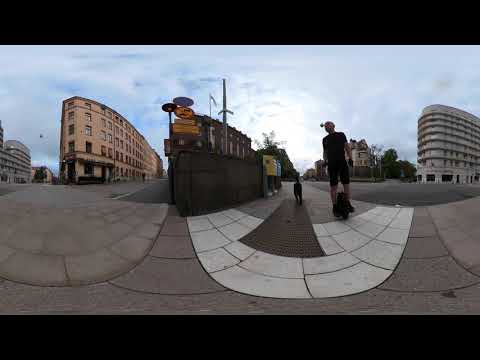The photograph captures a vibrant city scene taken from ground level outside on a clear day. In the foreground, a white male dressed entirely in black—wearing a black t-shirt and black shorts—rides a one-wheeled electric device, possibly a hoverboard, as a small black dog follows closely behind him without a leash. The man appears to be moving towards the camera along a curved street. 

Surrounding him are several distinctive buildings. To the right, there's a six-storied white building with a smooth, curved design. Flanking the center is a tall brown building approximately eight stories high and another white structure reminiscent of a ship’s prow, housing signage and a flagpole. Additionally, a smaller domed building and a taller white building are seen in the background. The sky is mostly blue, dotted with cirrus clouds, completing this dynamic urban tableau.